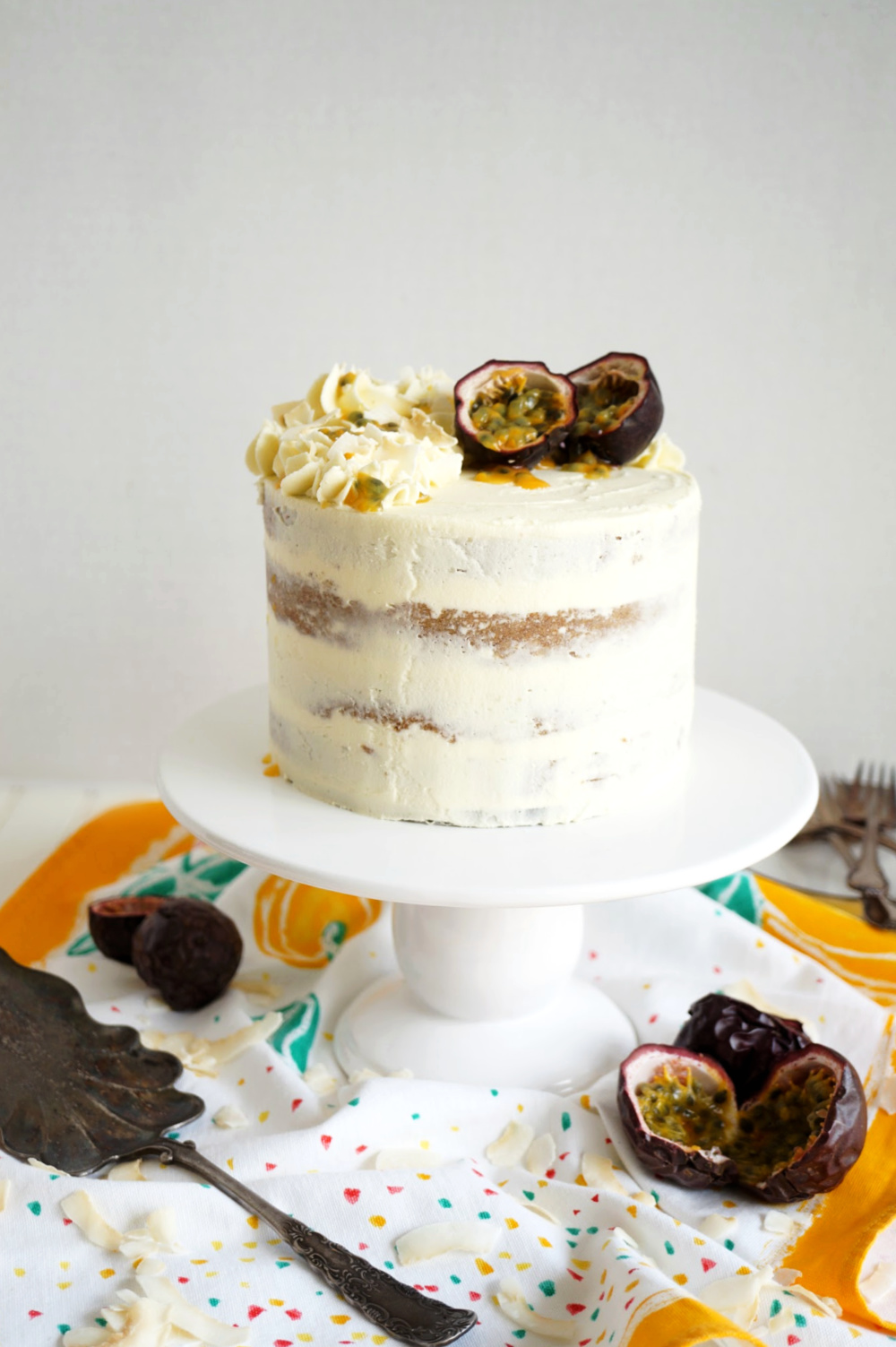The photograph showcases a beautiful, multi-layered cake elegantly displayed on a white cake stand. Frosted uniformly in white, the cake is topped with delicate puffs of cream and adorned with halved figs, their dark red, brown-tinged skins contrasting vividly with the bright green seeds inside. The cake stand is positioned on a festive white tablecloth speckled with colorful dots in red, yellow, blue, and green, adding to the celebratory feel of the scene. Surrounding the cake, halved figs are scattered across the tablecloth, providing a rustic touch. A cake spoon rests nearby, accompanied by forks in the background, ready for serving. The entire setup is framed against a neutral gray background, ensuring the vibrant colors and intricate details of the cake and fruit are the focal points of the image.